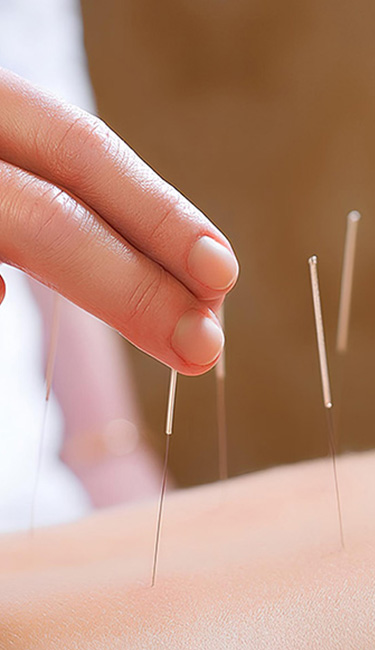This is a detailed, close-up photograph of a person performing acupuncture. The focus is on the intricate details of the human skin, where you can clearly see the pores and little hairs. Several acupuncture needles are inserted into the skin, each with a slim, long handle. Two fingers, showing clear wrinkles and fingernails, come into the image from the left, holding one of the needles. The individual performing the acupuncture is wearing a white outfit, and in the blurred background, there’s a person dressed in white with something indistinct around their wrist. The background features a dark, muted brown color, adding a contrasting backdrop that highlights the precise and serene act of acupuncture.